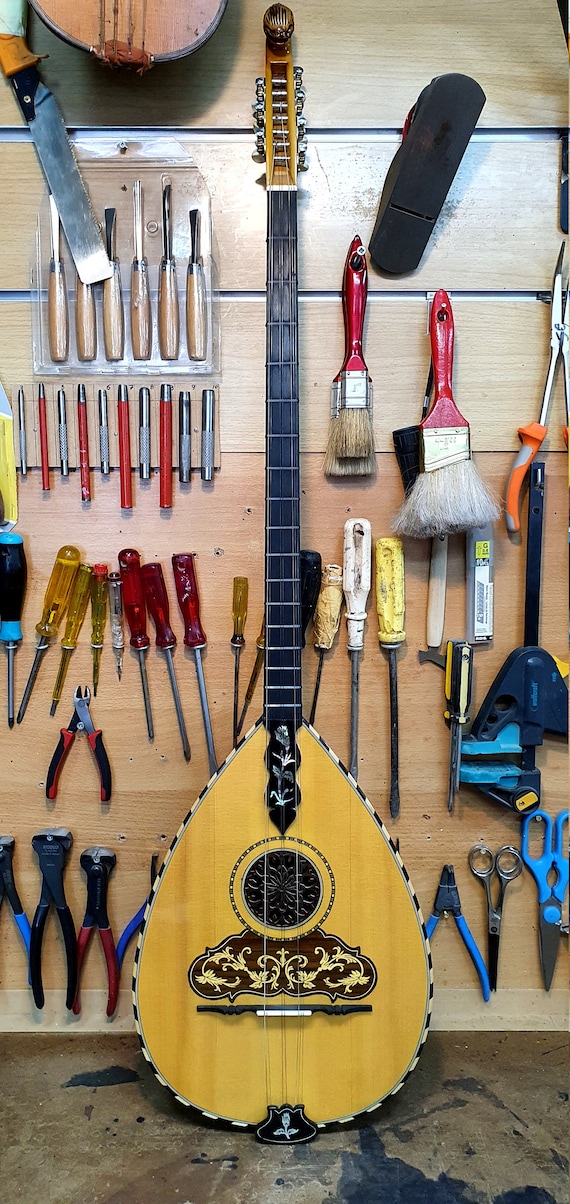The image showcases an organized array of various tools meticulously hung on a wooden, paneled wall. A collection of screwdrivers is grouped together, flanked by wire cutters, paint brushes, awls, and a diverse assortment of other tools. Adding a unique touch to the scene is a long-handled guitar leaning against the wall, its extended neck stretching up several feet, nestled among the tools. 

Above a section of the tools encased in plastic, only the bottom and strings of another guitar are visible, making its type indistinguishable. A tool hangs in front of this guitar, overlapping a set of tan-handled tools. The floor beneath this display is unfinished, with noticeable black paint spills contrasting against its brown surface.